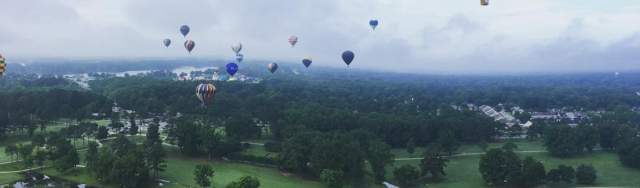In this expansive horizontal image, the vibrant scene is dominated by an array of colorful hot air balloons soaring gracefully in a grayish-blue, cloud-filled sky, suggesting a dedicated balloon event. Each balloon displays its own unique pattern, with prominent colors such as blue, white, red, and darker whites, filling the air at varying heights. The viewpoint appears to be from someone within another balloon, giving the impression of being on the same plane as these mid-flight marvels. Below this spectacle lies a verdant landscape, densely packed with lush, well-watered treetops, indicating a healthy ecosystem. Stretching out beneath the green expanse are hills with carefully tended greenery, reminiscent of a golf course, as well as a mix of buildings hinting at a small town on the right and larger structures approaching a mountain range in the left background. The scene captures the juxtaposition of tranquil nature and human habitation, unified under the serene ballet of floating balloons.